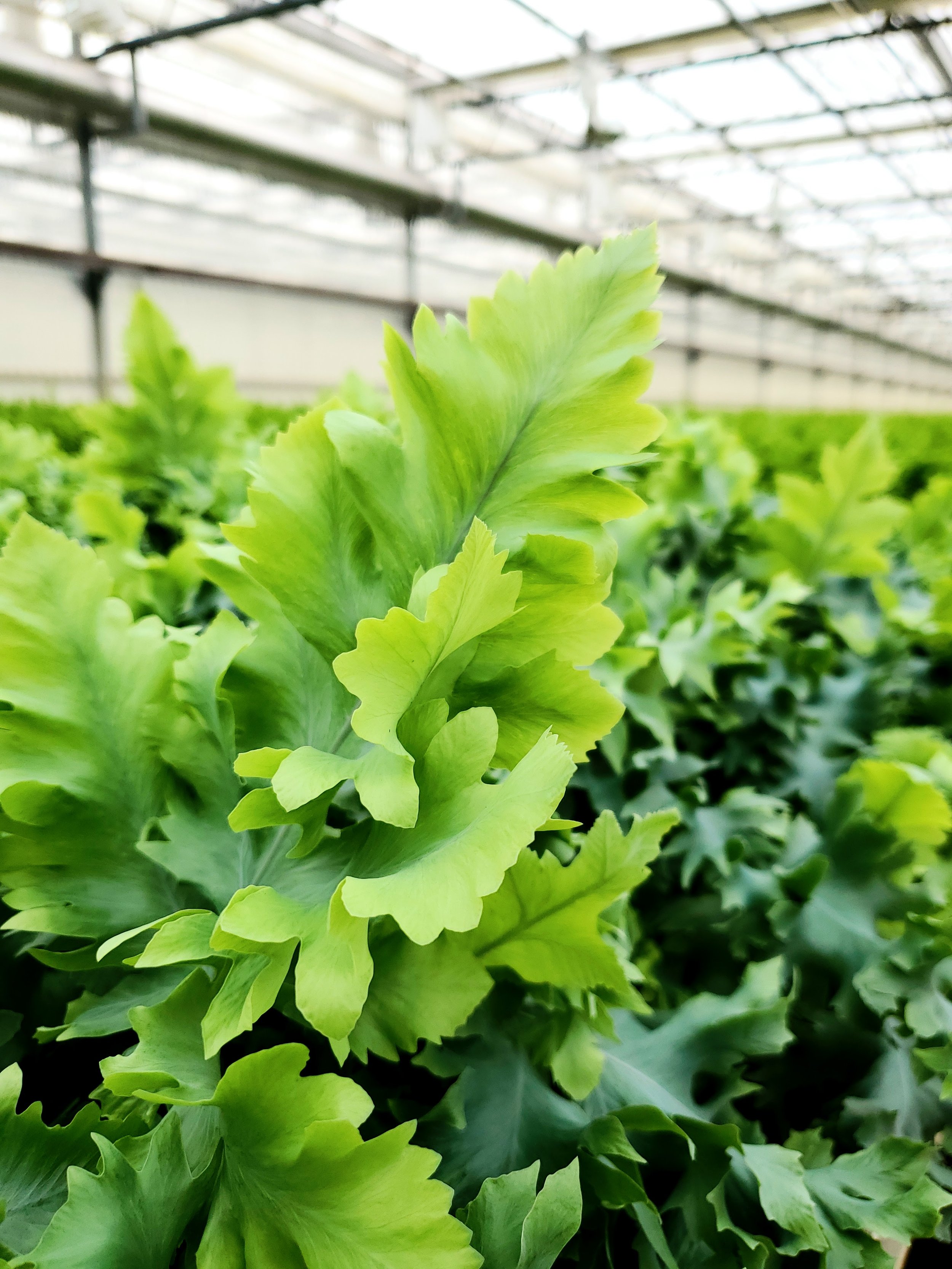In this detailed image, we are looking at a vibrant greenhouse filled with numerous green leafy plants, each displaying a variety of shades from light green to dark green. At the forefront, a plant with pronounced, curly green leaves stands out, capturing the incoming sunlight from above. The greenhouse structure features beige walls, ceiling windows that allow sunlight to filter through, and several silver metal frames supporting the walls, which some might describe as resembling garage doors. The roof appears to be made of black glass or plastic, creating a striking contrast as it allows beams of light to pour in and nourish the plants below. In the background, the plants blur into the distance, suggesting a lush, densely-packed environment. Additionally, there are hanging structures from the ceiling and intricate piping systems, likely for watering, that connect the glass panels. Overall, the image encapsulates a lively, sunlit greenhouse where the interplay of light and varying shades of green breathes life into the space.